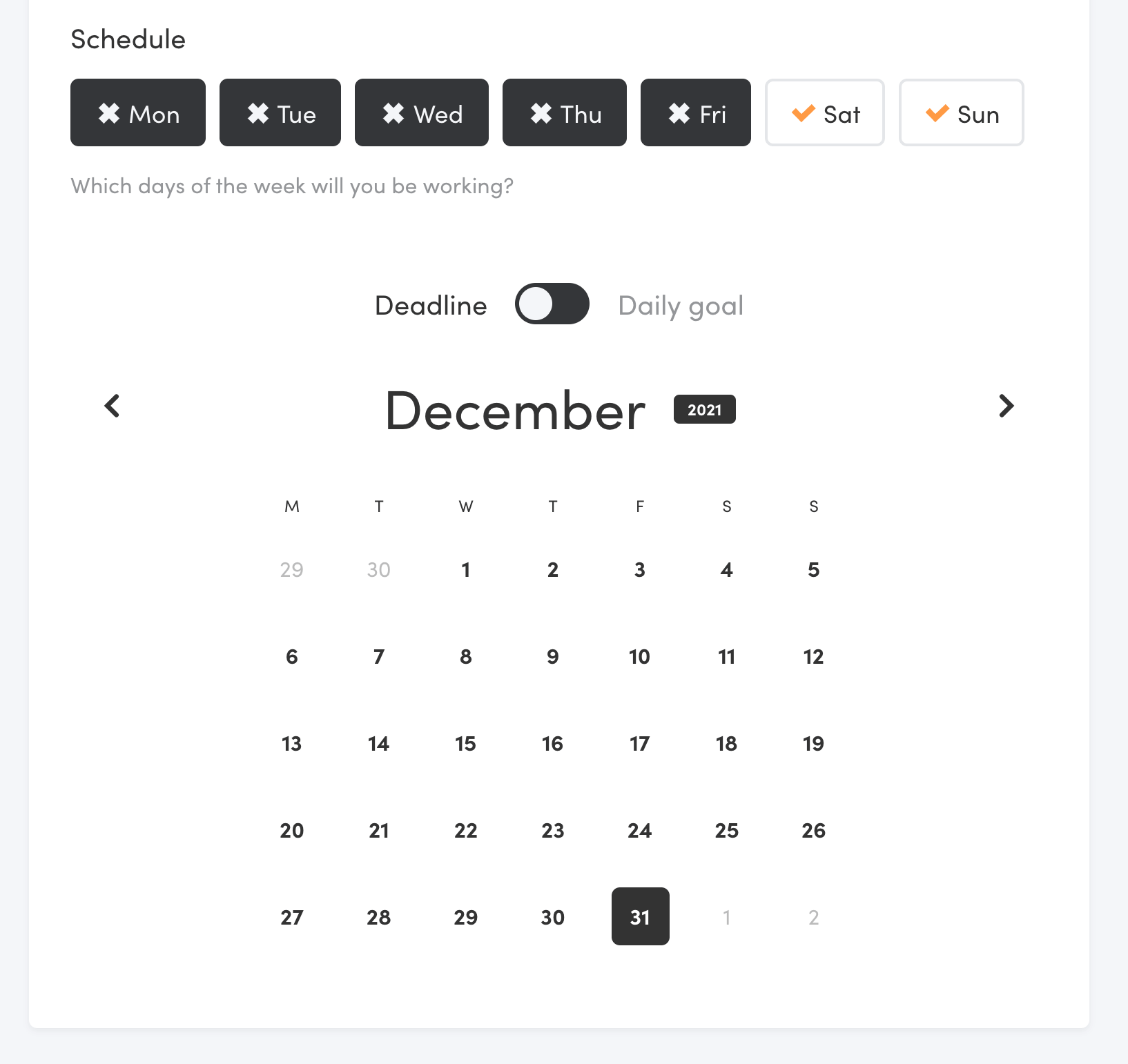The image features a light blue background encompassing the entire left, right, and bottom edges. Prominently displayed at the top is a schedule section with the text "Which days of the week will you be working?" Each weekday—Monday, Tuesday, Wednesday, Thursday, and Friday—is represented with black boxes containing white X marks. In contrast, Saturday and Sunday are depicted in white boxes with small orange checkmarks beside them. 

Below the schedule, the image presents a white section labeled "Deadline." This section includes a black toggle switch and a section for setting a daily goal. Adjacent to these elements, there are left and right arrows flanking the label "December" and a small black box containing "2021." Below this is a calendar for December, with the date 31st highlighted in a black box, indicating a special significance for that day.

Overall, the image is a well-structured, visually organized display detailing a weekly work schedule, deadlines, and daily goals, with a particular emphasis on December 31st.